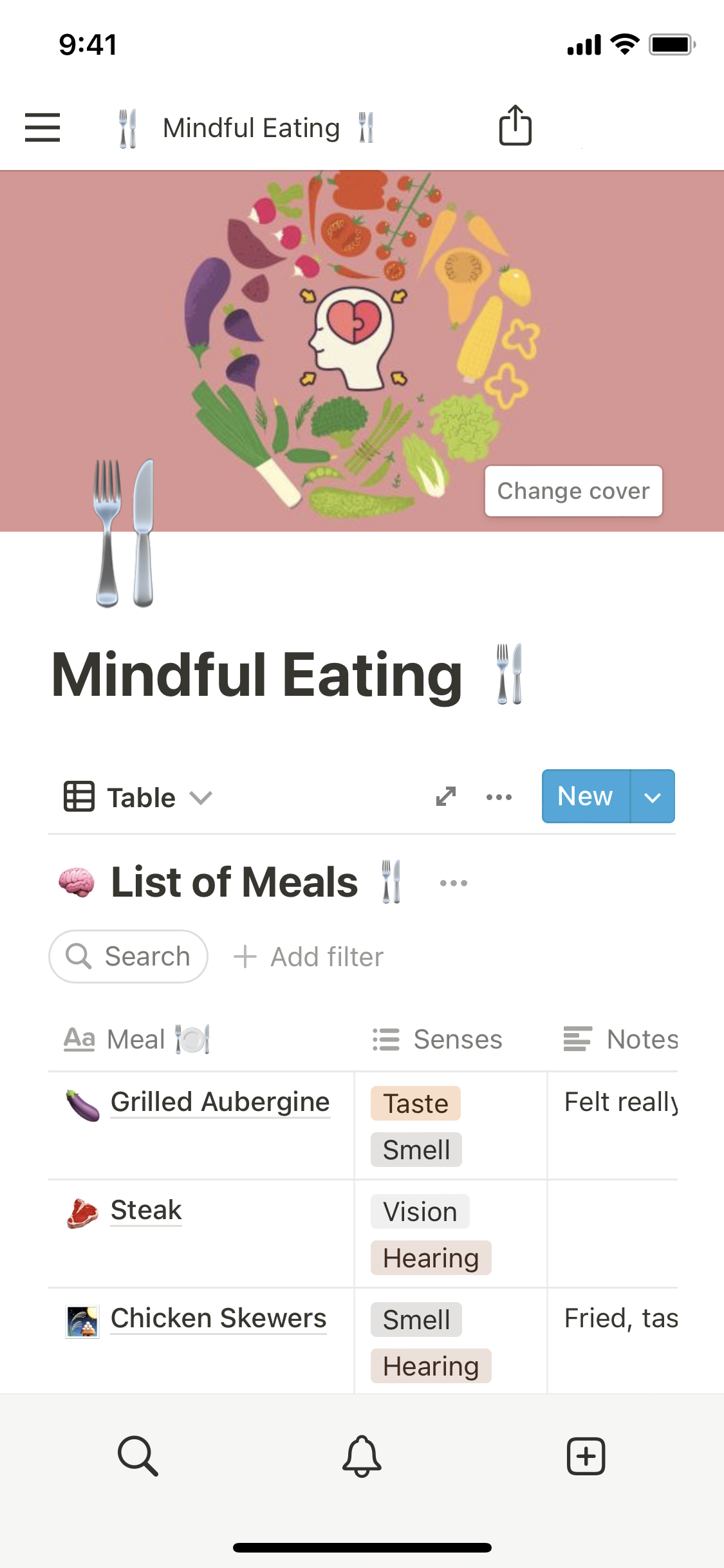At the top left corner, the time reads 9:41, while on the right side, the battery icon is nearly full, displayed as a black bar. Below this, the phrase "Mindful Eating" is prominently featured. To the left, there is an image of a fork and knife. In the center of the composition is a pink square containing an illustration of a person's profile with a red heart inside. Surrounding this central image are various colored sections: a purple area with eggplants and grapes, a red area featuring tomatoes, a yellow zone showcasing corn, an orange section with carrots, a light green area with lettuce, and finally, a darker green section appearing to display kale. Below this, the fork and knife reappear with the words "Mindful Eating" and "Table" underneath. Below "Table," there is a list of meals accompanied by a search bar. The list includes "Grilled Aubergine" with an image of an eggplant beside it, "Steak" with a small red steak icon, and "Chicken Skewers." To the right of the "Chicken Skewers" entry are the words "Smell" and "Hearing."